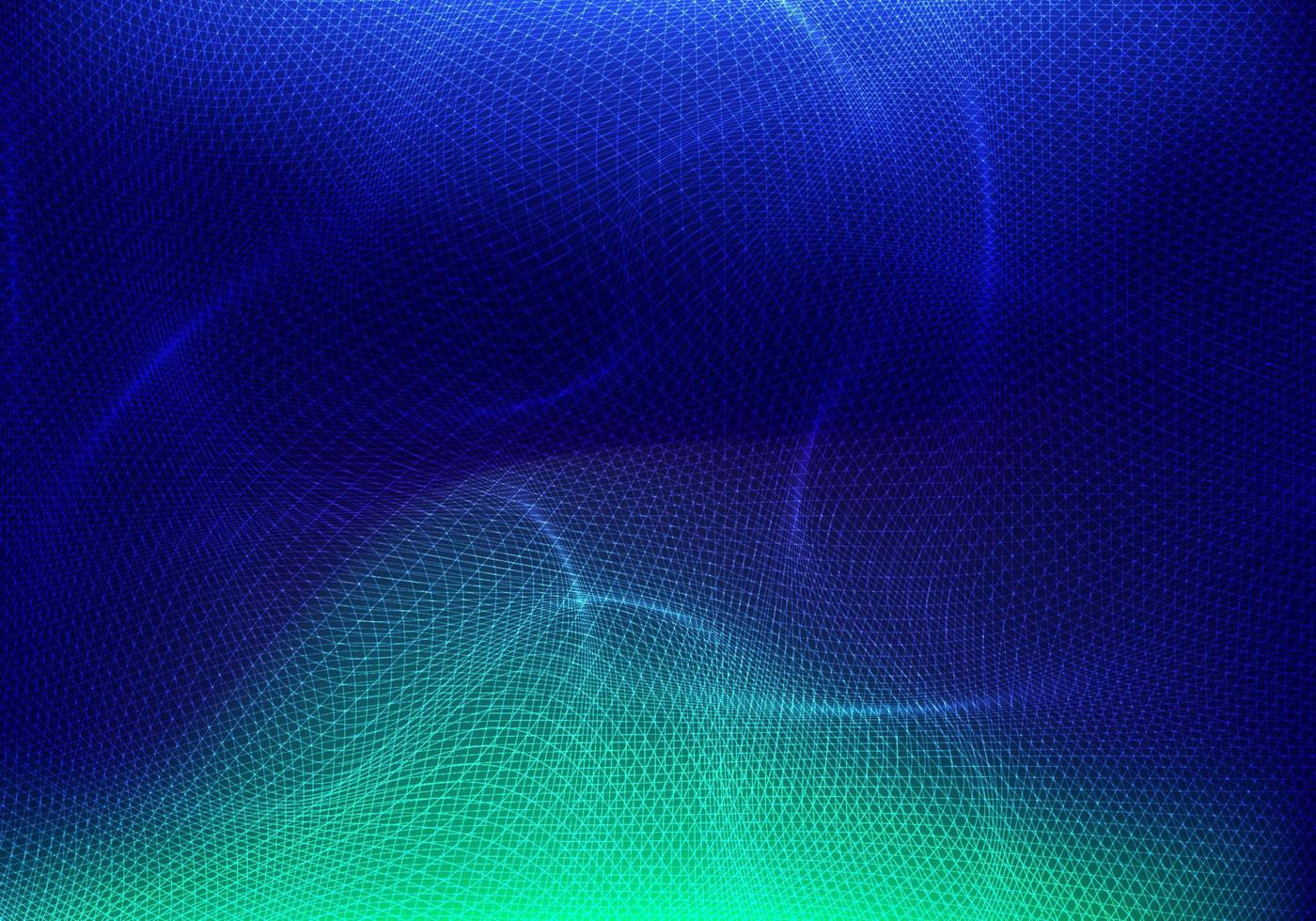The image features an intricate network of countless intersecting lines emanating from every corner and edge, creating a blend of straight, curved, and wavy patterns that imbue the image with a dynamic and almost three-dimensional effect. The top half of the image transitions from a bright blue at the edges to a deeper, almost purple hue towards the center, while the bottom half shifts from a teal to a vibrant lime green, with the darkest tones residing in the corners. Thin, bright lines crisscross the composition, occasionally forming shapes reminiscent of diamonds, S's, and parentheses, adding to the complexity. The coloration and linework fuse together seamlessly, giving the impression of an intricate digital creation designed to captivate and confuse the eye.